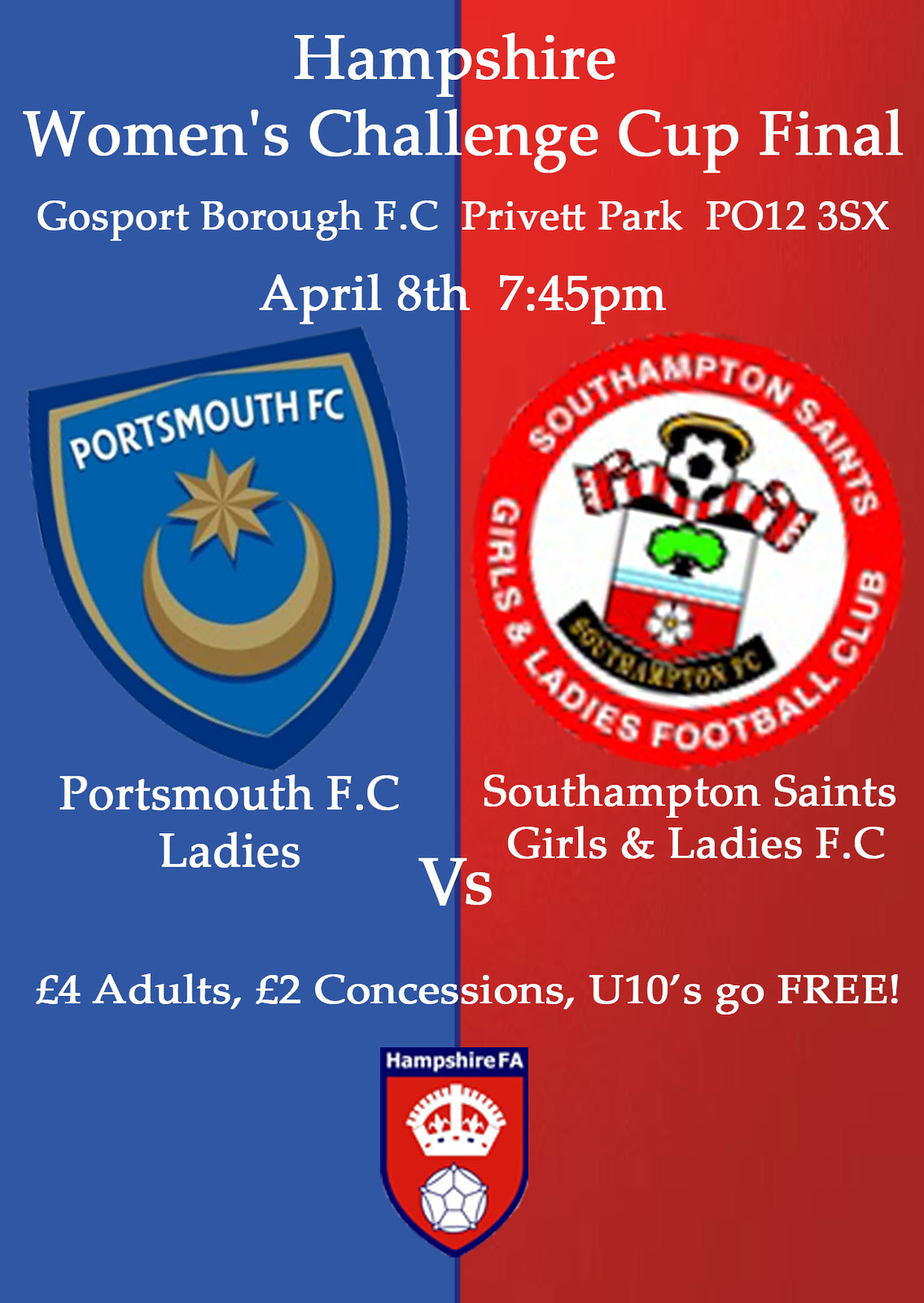The poster for the Hampshire Women's Challenge Cup Final is split into two distinct sections. The left side features a blue background and the right side a red one. At the top, it prominently displays the event details in white text: "Hampshire Women's Challenge Cup Final. Go Sport, Borough FC, Privet Park, P.O. 123SX, April 8th, 7:45 p.m." 

Beneath these details, the left side showcases the logo of Portsmouth FC Ladies, marked by a blue-edged seal with the text "Portsmouth PFC" at the top, and a gold star and crescent moon below. The right side presents the logo for the Southampton Saints Girls and Ladies Football Club, which consists of a red-edged circle featuring a crest with green trees, a flower, a red and white striped scarf, and a soccer ball.

Below the team logos, the competitors are noted: Portsmouth FC Ladies versus Southampton Saints Girls and Ladies FC. The bottom part of the poster states the ticket prices: Adults £4, Concessions £2, and free entry for under 10s. Additionally, the Hampshire FA logo, featuring a crown and a starfish design, is positioned at the very bottom of the poster.